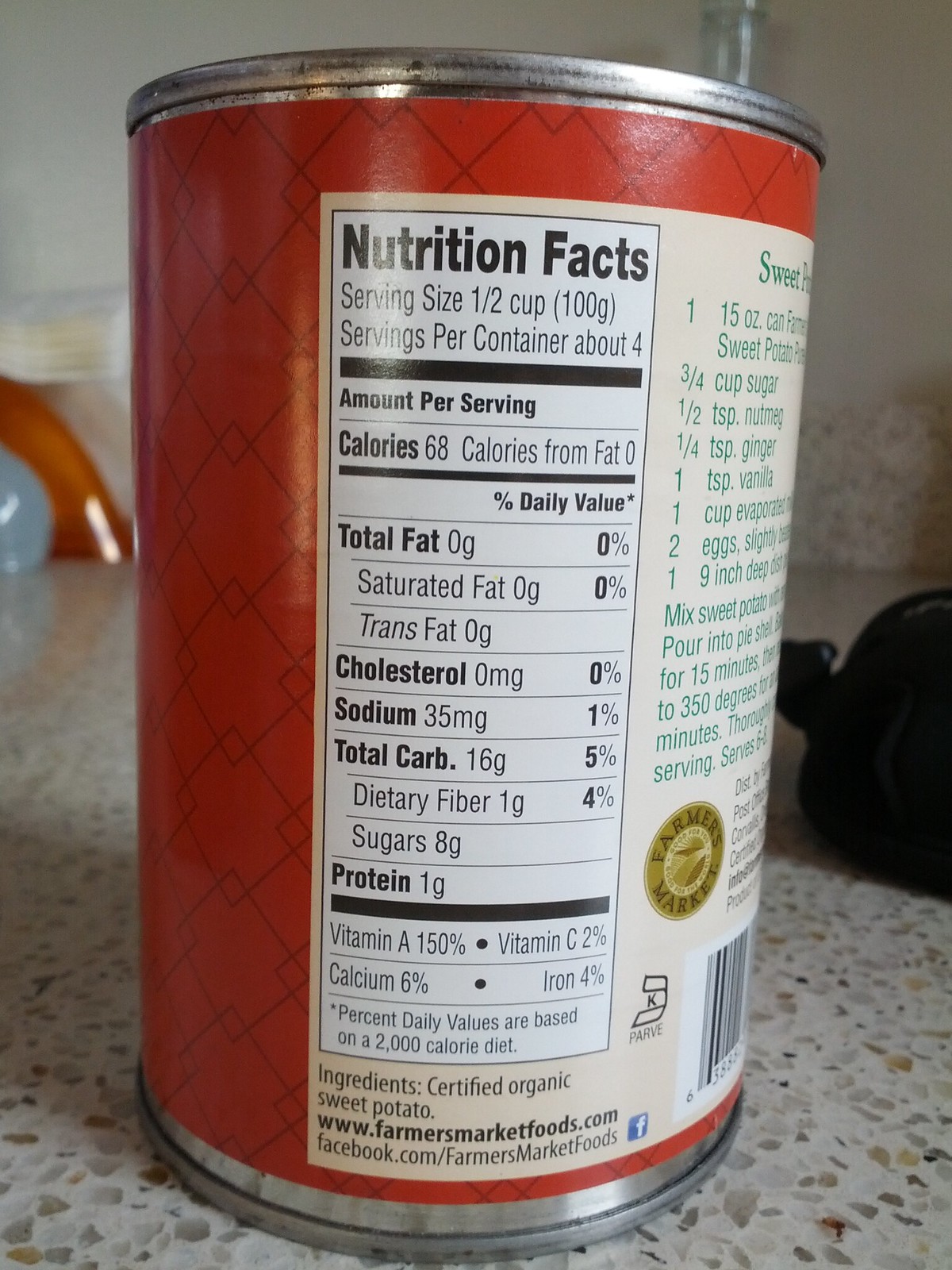The image depicts a can of food prominently displayed on a multi-colored terrazzo countertop, speckled with brown and gray spots. The can, featuring a red label with a black grid pattern and a gold "Farmer's Market" logo, lists its nutrition facts on a white section of the label. The can's nutritional information is detailed as follows: serving size is half a cup (100 grams), with approximately four servings per container. Each serving contains 68 calories, with zero calories from fat. The breakdown includes zero grams of total fat, saturated fat, and trans fat; zero milligrams of cholesterol; 35 milligrams of sodium (1% of the daily value); 16 grams of total carbohydrates (5% of the daily value) including 1 gram of dietary fiber (4% of the daily value) and 8 grams of sugars. It also has 1 gram of protein. Notably, it provides 150% of the daily value for Vitamin A, 2% for Vitamin C, 6% for Calcium, and 4% for Iron. The ingredients listed are certified organic sweet potato. A URL, www.farmersmarketfoods.com, and a Facebook link are also indicated on the label. Additionally, there appears to be a recipe on the opposite side of the label.